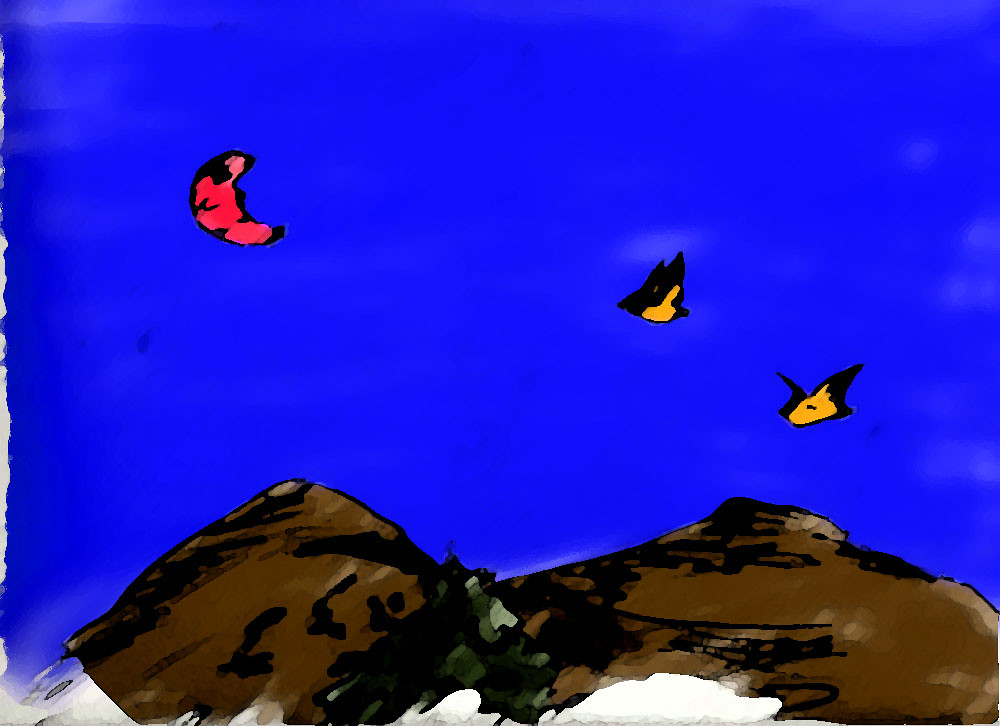The image is a digitally created composition with a landscape orientation featuring a predominantly blue background, evoking an ambiguous scene that could either represent an underwater domain or a vast, rich blue sky. In the blue expanse, two yellow and black-winged creatures drift on the right side, resembling birds or butterflies without clearly defined features. Towards the top left corner, a striking red, banana-shaped form with a black outline appears, floating in a manner that adds to the ambiguity of the setting. The lower third of the image showcases two brown, roughly sketched mountains with darker peaks, possibly embellished with black and green details that might represent trees or rocks and seaweed if seen underwater. Sporadic white smudges and patches, along with incomplete blue sections, create an unfinished impression. Moreover, a crescent moon in reddish and black hues appears subtly on the left side, enhancing the enigmatic quality of this scene.